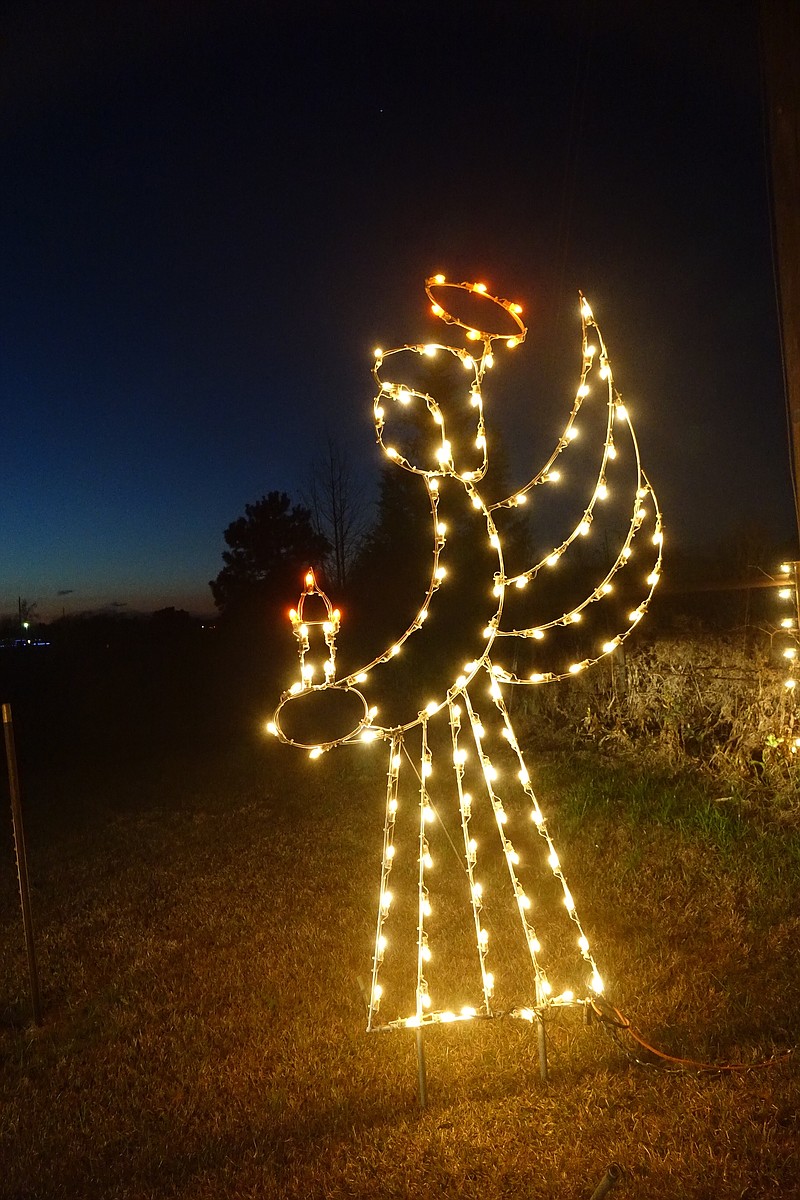The photograph, taken outdoors in the early evening, captures a vertically aligned rectangular image of a Christmas lawn ornament shaped like an angel. Lit up against the darkening sky with hues transitioning from black at the top to a darker blue towards the middle left, the angel stands prominently in the center. The angel, highlighted by white lights, features an illuminated red halo, and holds a red-tipped candle in outstretched hands. Its simplistic, almost clipart-like design is secured to the ground by two to three metal stakes, and there is a visible wire extending from it, suggesting it is plugged in. At the bottom of the image, patches of grass are visible, giving way to taller grass and possibly a field on the right. An additional, partially visible lawn decoration adorned with similar lights can be seen near the taller grass. The background additionally shows faint silhouettes of trees and even a few stars twinkling in the night sky.